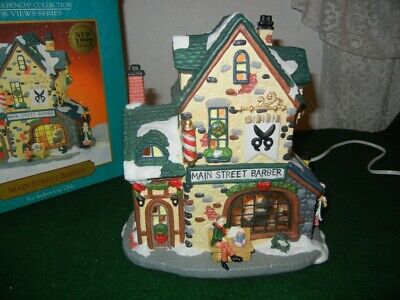This photograph features a detailed model from a traditional Christmas village set. The centerpiece is a yellow cobblestone building with a distinct green pointy roof topped by two chimneys, adorned with patches of snow. Dominating the front facade is a green-bordered sign with black text that reads "Main Street Barber" on a white background. Below this prominent sign is an arched window, and situated in front of it is a yellow bench. Seated on the bench, a man dressed in a green jacket and red scarf adds a touch of life to the scene. The left side of the building includes a door decorated with a festive wreath. The model stands on a cement or rock gray base, also partially covered in snow. In the background, the building’s packaging is visible, featuring an image of the model itself. A cord emerges from the back of the building, hinting at internal lighting. This comprehensive model is a quintessential element of a Christmas village display, combining architectural charm with seasonal decoration.